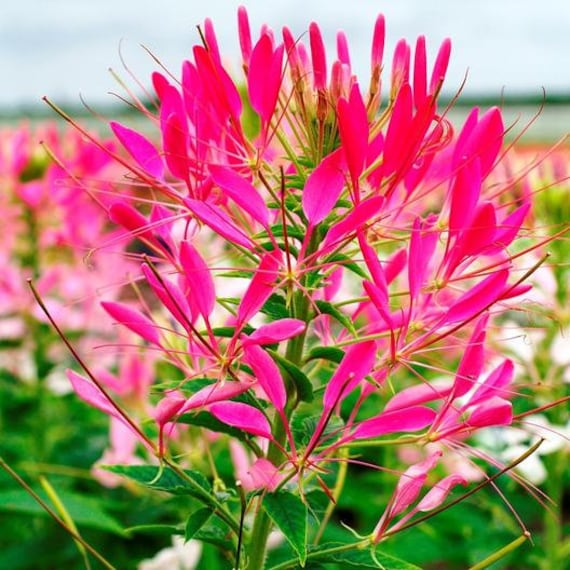In this image, we see a striking photograph featuring a cluster of vibrant pink flowers that immediately capture attention. The most prominent flower, with its vivid pink petals, stands out prominently against its lush green leaves and stem. Surrounding it, we notice other flowers in hues of pink and white, adding to the overall bouquet's charm. The background of the image showcases greenery and is set against a partly cloudy sky, featuring shades of white and blue. In the distant horizon, a body of water, possibly a lake, is visible, reflecting a serene blue. The composition beautifully contrasts the vivid pink flowers with the tranquil landscape, making the photograph exceptionally captivating. The cluster consists of approximately 20 to 25 flowers, contributing to a full and vibrant visual experience that stands out brilliantly against the green foliage and the expansive sky.